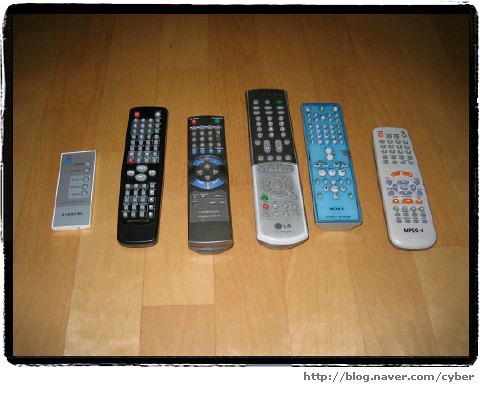The image showcases six distinct remote controls lined up horizontally on a blonde maple wood floor, which may be either laminate or real maple hardwood. The photo is framed with a rounded black outline, reminiscent of a tablet computer. Starting from the left, the first remote is a small, light gray or white one, possibly for a fan, featuring very few buttons. Next is a long, standard black TV remote followed by a gray TV remote. The fourth remote has a dual-colored body with its bottom half potentially covered in protective film or naturally white, and the top half in black. The fifth remote stands out with a blue, potentially protective film coating and has a very rectangular shape with sharp corners. The final remote is white, bearing a name that's not clearly legible, and adorned with several colored buttons. All remotes differ in size, make, and model, and are simply placed side by side on the floor. Below the framed image, the URL "http://blog.navernaver.com/" is visible.